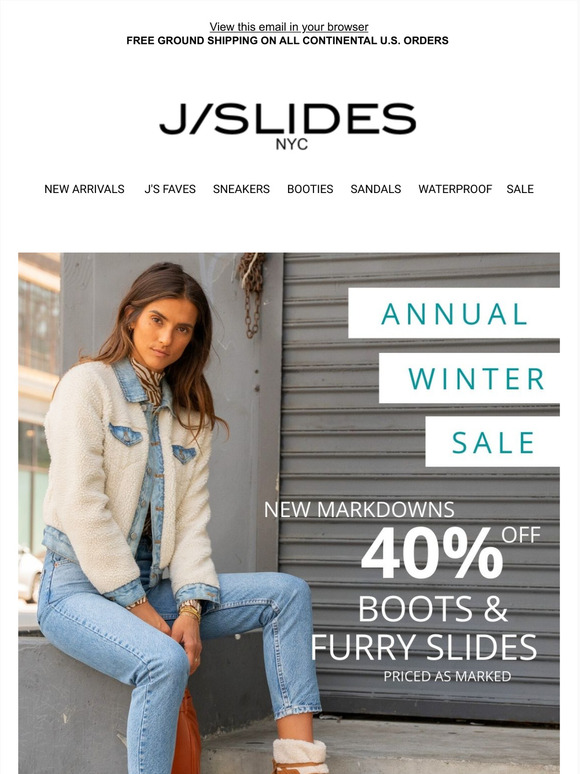### Detailed Caption:

**Digital Advertisement for JSLIDES NYC**

This nearly square, rectangular digital advertisement by JSLIDES NYC features a minimalist design with a very thin light gray border. At the top of the ad, there is a clickable, underlined text saying, "View this email in your browser."

Directly beneath, a bold announcement in all caps reads, "FREE GROUND SHIPPING ON ALL CONTINENTAL U.S. ORDERS."

Following this statement is a section of blank white space, ensuring the text stands out starkly. At the center, the brand name JSLIDES stretches across, with the capital 'J' followed by a backslash and the word 'Slides.' Below this, in smaller caps, it says, "NYC," indicating the brand's connection to New York City.

Inline with the brand name is a row of clickable categories, each in small capitals. These categories include: New Arrivals, Jay's Faves, Sneakers, Booties, Sandals, Waterproof, and Sale, suggesting a variety of footwear options.

The focal point of the ad is a large square photograph of a model sitting on a short gray concrete wall. The setting appears to be urban, with a gray concrete background and a corrugated metal door, reminiscent of a security or garage door found in New York City. In the upper left part of the image, a glimpse of a building confirms the outdoor location.

The model wears blue jeans paired with a distinctive jacket made of white fleece and trimmed with blue denim on the cuffs, collar, front placket, and pockets, harmonizing with her jeans. Beneath the open jacket, she sports a high collared shirt. She sits with her arms between her legs, holding a leather pocketbook, and wears mid-shin height boots, though only her left boot is visible.

Overlaying the photo is a promotional message for the "ANNUAL WINTER SALE," styled in teal all-caps text on progressively smaller white bars resembling a sideways bar graph. Beneath, in bold white lettering, it announces "NEW MARKDOWNS 40% OFF." The "40%" is notably oversized and bolded to catch the reader's eye. It concludes with "Boots and Furry Slides, priced as marked."

This enticing ad is designed to draw attention to the seasonal sale and highlight new markdowns, encouraging customers to explore the discounted selections of boots and slides.